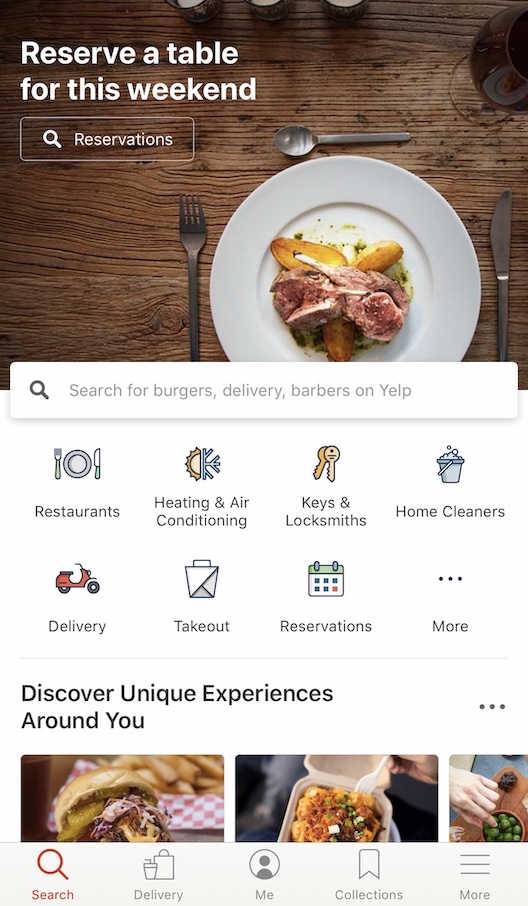**Detailed Caption:**

Captured within this image is a screenshot of a phone display featuring a mobile app interface, set against the background of a rustic, well-used wooden table typical of a restaurant setting. Prominently displayed on the screen is a white box prompting the user to "Reserve a table for this weekend" with an embedded option to make reservations.

In the scene, resting on the wooden table is a tantalizing display of food: a neatly arranged white plate featuring savory sausages accompanied by a variety of vegetables. Flanking the plate are pristine silverware, with a knife positioned on the right and a fork on the left, while a spoon rests on top of the plate, underscoring the readiness for a delightful meal.

Further, the interface contains actionable text encouraging users to "Search for burgers, delivery, and barbers on Yelp."

Behind the primary prompt, the rest of the interface is showcased against a clean, white background. A section labeled "Restaurants" includes a search function accompanied by a restaurant icon, and subsequent searchable categories such as "Heating and Air" (with a corresponding icon), "Keys and Locksmith" (depicted with a set of keys icon), "Home Cleaners" (represented by a bucket full of soap bubbles), "Delivery" (illustrated with a small car icon), "Takeout" (shown with a cardboard box icon), "Reservations" (marked by a calendar icon), and an option for "More."

Below these categories, the app invites the user to "Discover unique experiences around you," showcasing appetizing images of various takeout options. These include a delicious burger served with French fries, possibly featuring pulled pork and coleslaw, a takeaway container filled with shrimp, green onions, and assorted vegetables, and a final image displaying a refreshing bowl of fresh green peas.

This informative and visually engaging interface aims to enhance the user's dining experience by providing easily accessible features for discovering and reserving at local eateries.